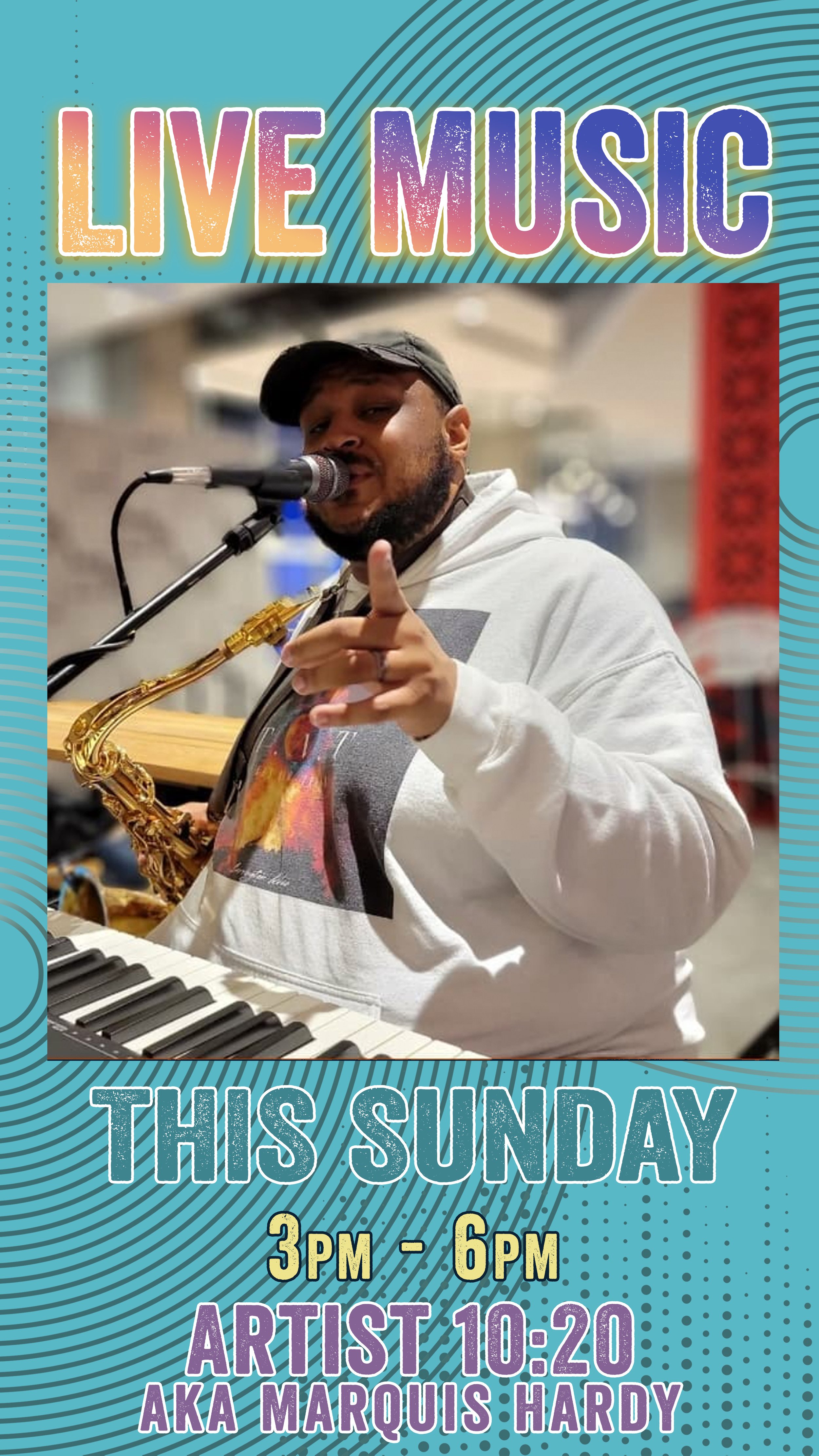The digital flyer for the concert features a teal background adorned with a darker teal thumbprint pattern. Dominating the top of the flyer is the phrase "Live Music," showcased in a vibrant gradient featuring yellow, pink, and purple hues. Central to the design is a photograph of a heavyset African-American man who commands attention with his white hoodie and black baseball cap. He sports a beard and is energetically pointing at the viewer while speaking into a microphone. Around his neck, he wears a strap holding a saxophone, and in front of him lies an 88-key keyboard. Below this engaging scene, the flyer details the event's timing: "This Sunday 3 p.m. to 6 p.m." The artist is introduced as "Artist 1020 aka Marquise Hardy." The design elements, including the swirling lines of the background, help to frame this compelling image of a modern musician.